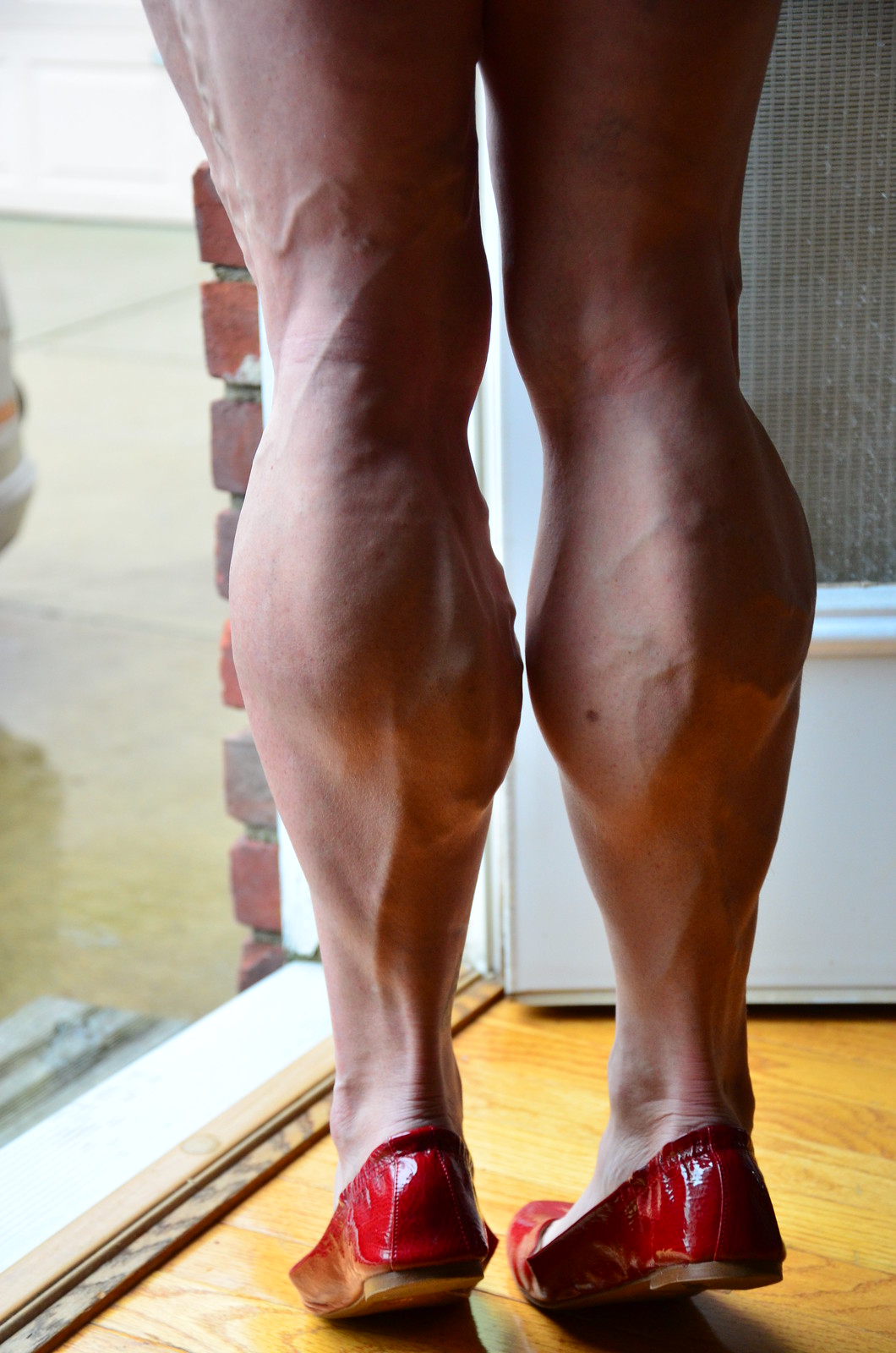The image depicts the lower half of a person's body, viewed from behind, showcasing their muscular, veiny legs standing on tiptoes. The person's fair-skinned legs are noticeably veiny and freckled, with one prominent freckle visible on the right leg. The legs appear strong and well-developed, with pronounced calf muscles and an irregular, lumpy texture due to the visible veins. The individual is wearing bright red, patent leather-like ballet flats with a slight heel and elastic around the opening. They are standing on a light brown, natural-colored hardwood floor in front of an open white door that features a window. The door frames an entrance leading outside where red brick siding can be seen on the left, along with a gray stair ledge and a shiny, wet cement driveway. The overall setting suggests an inside-to-outside perspective, highlighting the white door and frame, contrasting with the external brick and cement environment.